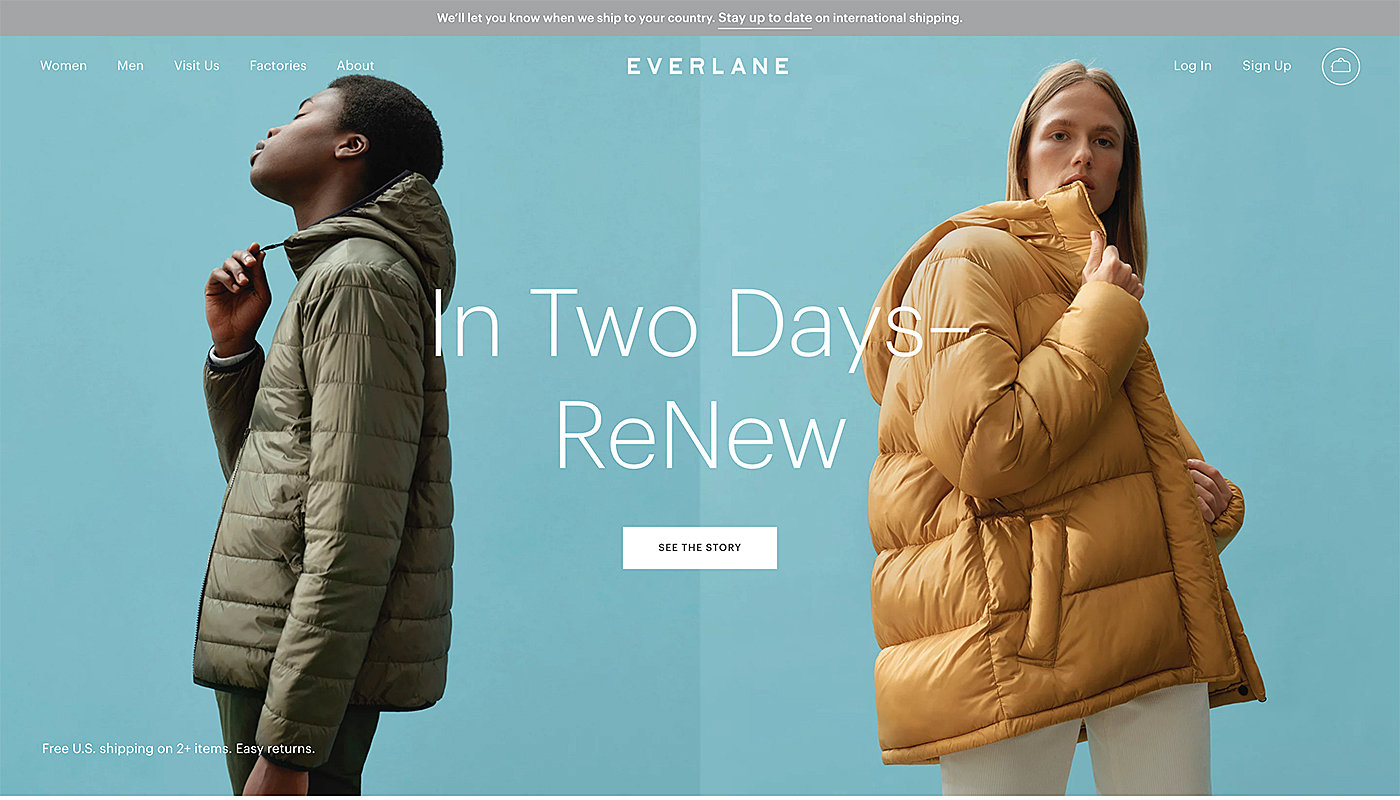This screenshot captures a web page from Everlane. At the top, a gray bar displays the message: "We'll let you know when we ship to your country. Stay up to date on international shipping." Below this, the Everlane logo is set against a seafoam-colored background. 

Prominently featured are two models: a Black male with short black hair on the left, and a white woman with long blonde hair on the right. Both are adorned in heavy winter coats; the man wears a gray coat and is turned sideways, while the woman, in a brown coat, faces the camera but has her body turned sideways.

In white text between the models, it reads: "In two days – renew." Just beneath this, a white button invites viewers to "See the story." At the bottom left of the page, another message announces: "Free US shipping in two days, easy returns." 

The overall page showcases Everlane's winter outerwear collection, highlighting the shipping options and return policies for U.S. customers.